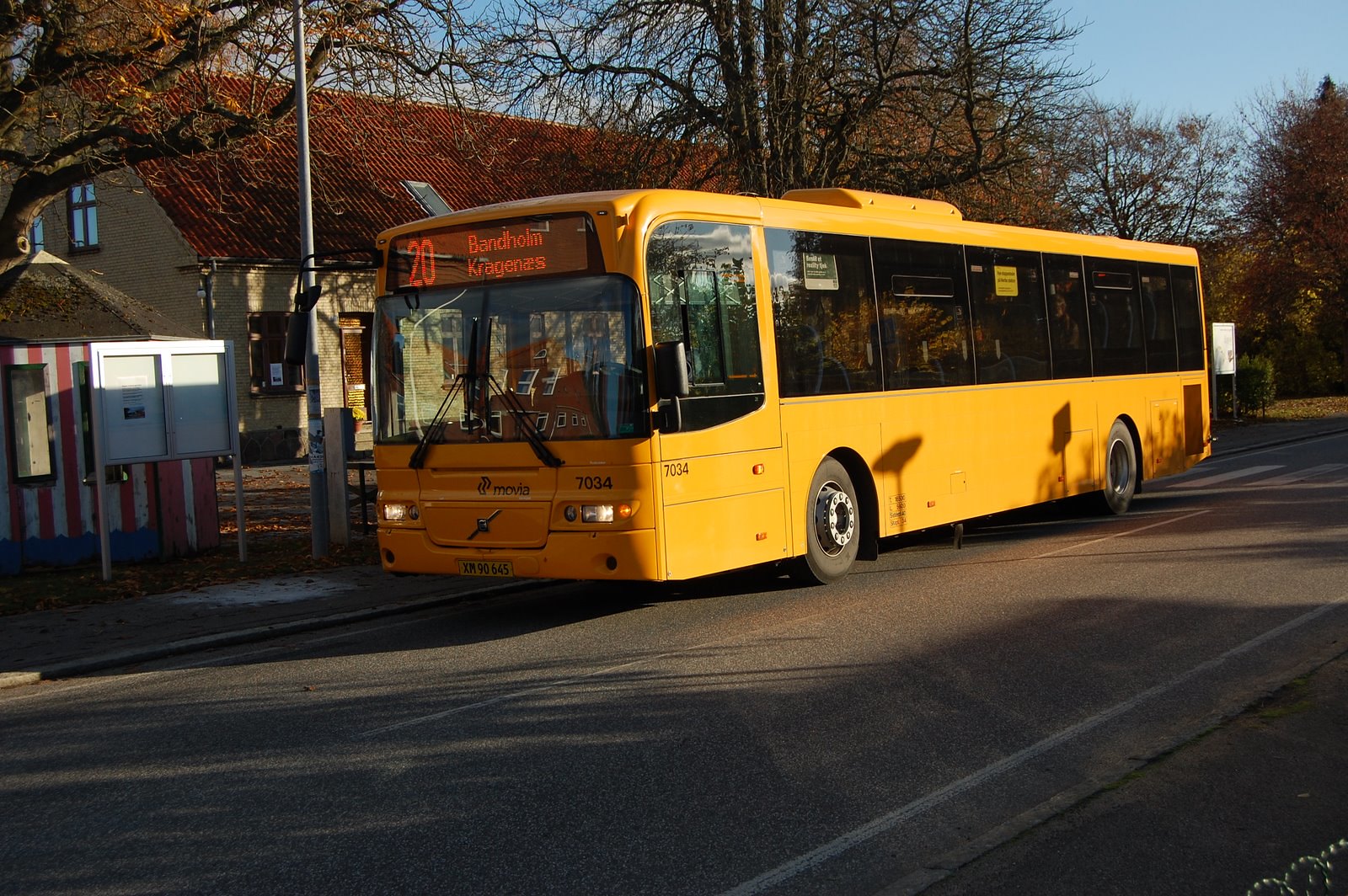A bright canary yellow city bus is prominently featured in the image, stopped at a bus stop on a clean, paved street with white dashed center lines. The bus, identified as number 20 on its digital display above the windshield, has large, tinted windows and is marked with the number 7034 on its side. The headlights are on, and black windshield wipers extend towards the center of the large front window. To the left of the bus, there is a silver signboard without any text.

In the background, various buildings can be seen. One has red and white horizontal stripes, while another features a reddish roof with visible windows and a skylight. The scene is set likely in late autumn or early winter, as the trees are mostly bare or have very few leaves clinging to their branches. The sunlight is casting long shadows across the scene, suggesting the photo was taken in the morning or late afternoon.